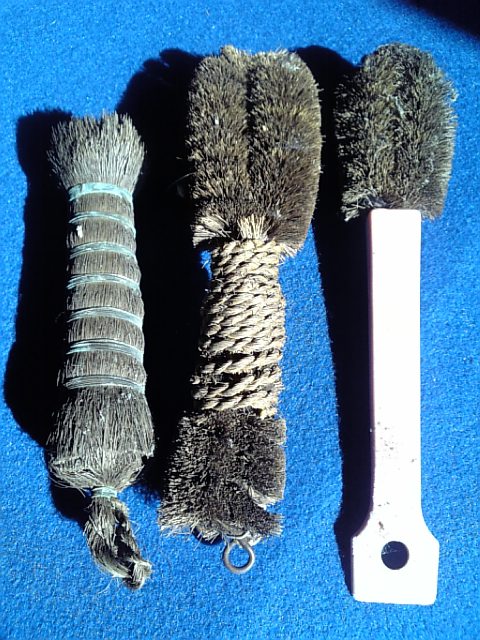The image depicts three different cleaning devices laid out on a textured light baby blue backdrop that resembles a towel. The first device on the left features stiff, tightly wound gray bristles with silver circles wrapping around its midsection, ending in a braided and closed base. The second device in the middle also showcases stiff, straight gray bristles woven together in the middle with a tan rope, complete with a metal hook protruding from its base. The third device on the right has a long rectangular handle, potentially made of either plastic or wood, though the shiny, poor-quality photo makes it hard to discern. This handle culminates in a gray bristled brush that somewhat resembles a microphone. Despite the subpar image quality, it's clear that all three items are intended for cleaning purposes.